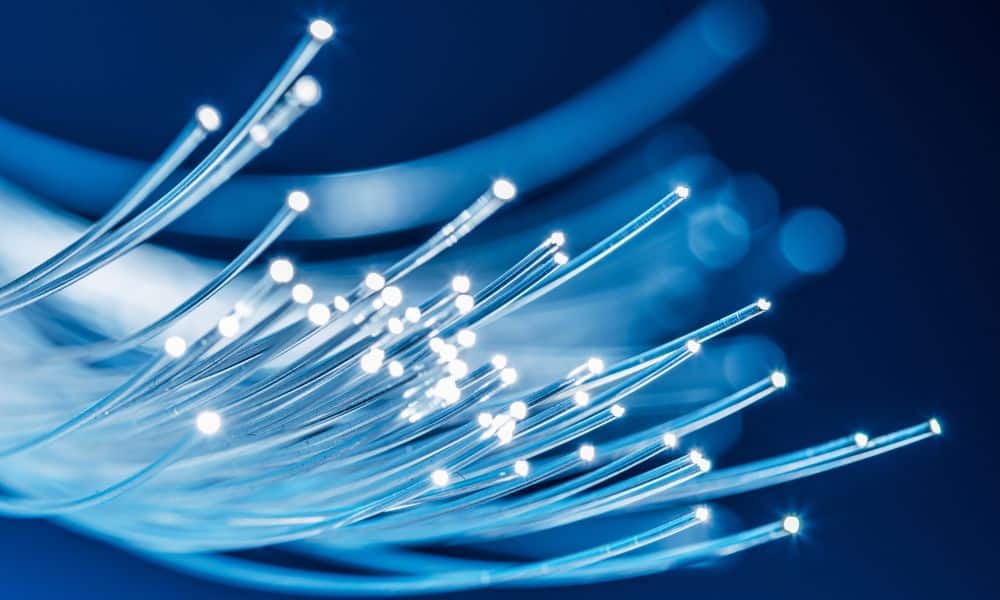This color photograph captures an artistic array of thin, silver, monofilament-like wires resembling optic fibers, which emerge from the bottom left and curve slightly upwards as they extend to the right. These wires, numbering over fifty, end in flat, clean-cut tips that shine brilliantly under the light, each tip glowing with a circular white gleam. The arrangement of the wires is random, with slight variations in their bends, creating an organic yet luminous display. The background transitions from a lighter blue on the left to a dark midnight blue on the right, featuring blurred, out-of-focus wires that add depth and contrast to the composition. There are no people or texts in the image, allowing the illuminated tips to dominate the dark blue gradient backdrop, enhancing the ethereal and futuristic feel of the photograph.